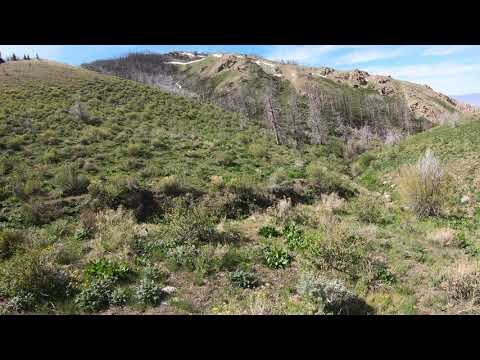The image is a photo framed by long black bars along the top and bottom, creating a letterbox effect. It features a verdant landscape with rolling hills and a prominent mountain. A hill rises from the right side to the top left, covered in lush green foliage, with sparse bushes and occasional trees, particularly concentrated on the left side. The right side reveals another hill rolling up from behind the first hill toward the top right of the image, also covered in greenery. Dominating the background, a large rocky mountain stretches nearly to the top of the image, contrasting with the greenery of the hills. Scattered across the ground are patches of brown and tan, highlighting cleared areas amidst the foliage. The sky above is a clear blue, adorned with wispy white clouds, adding to the scenic beauty of the landscape.